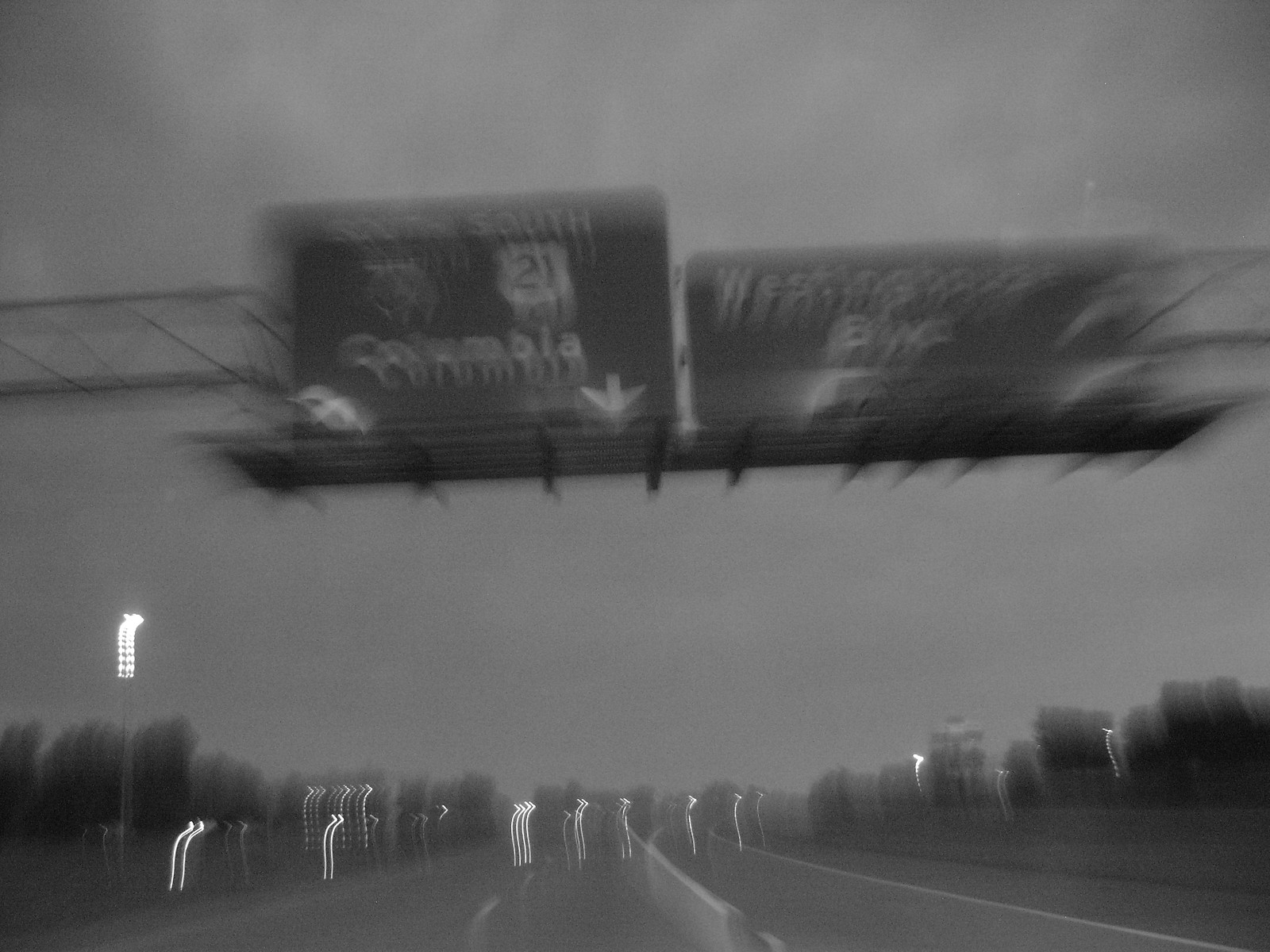A motion-blurred photograph captures the view from inside a moving vehicle driving down a highway. The image, evidently taken while in motion, shows a median wall to the right, dividing the lanes. Streetlights line both sides of the highway, with a particularly tall street lamp visible on the left. Overhead, green highway signs are suspended on long metal bars. The larger green sign on the left displays "South 77," "South 21," and "Columbia," with two white arrows pointing downward. Adjacent to it, another sign indicates "Westinghouse Boulevard," also accompanied by two white arrows directing traffic. The blurred elements underscore the speed and movement of the vehicle.